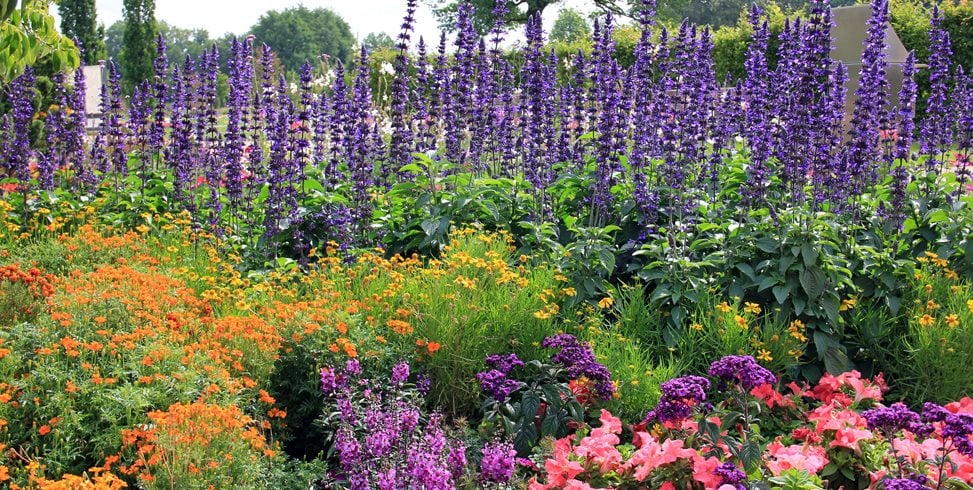This image is a vibrant, close-up shot of a bountiful and colorful garden, possibly a botanical garden. Dominating the scene are tall, vertical stalks of deep purple flowers that command immediate attention at the center. Surrounding these are a lush array of green leaves in various shades, interspersed with a vivid assortment of flowers in orange, yellow, pink, red, and lilac. The flowers cover the entire frame, creating a densely packed, almost bush-like appearance without any clear separation between individual blossoms. In the background, tall green trees frame the scene, and the sky above is a light, indistinct white. Subtly visible on either side of the image are gray structures, offering a hint of a boundary or surrounding environment. The diverse colors and tightly clustered blooms create a mesmerizing tapestry of floral beauty.